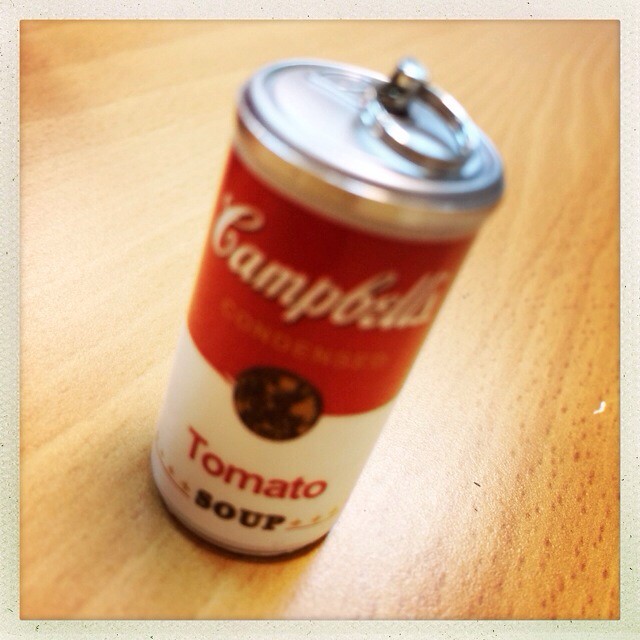This is a detailed photograph of a Campbell's tomato soup can, captured up close on a light wooden table. The image is bordered by a grayish frame, highlighting the central object. The can, unopened and metal, features the iconic red and white label with the traditional gold scrollwork and the word "Campbell's" in cursive at the top. The design includes a black circle within the red and white sections of the label and the word "condensed" near the bottom. Notably, the can functions as a keychain, with a key ring attached to its top. The photograph is focused on the texture and design of the wooden table, and the light reflecting off it, causing the can to appear slightly blurry due to its proximity to the camera. Although the can closely resembles the classic soup container, it is indeed a miniature, thin, key ring accessory.